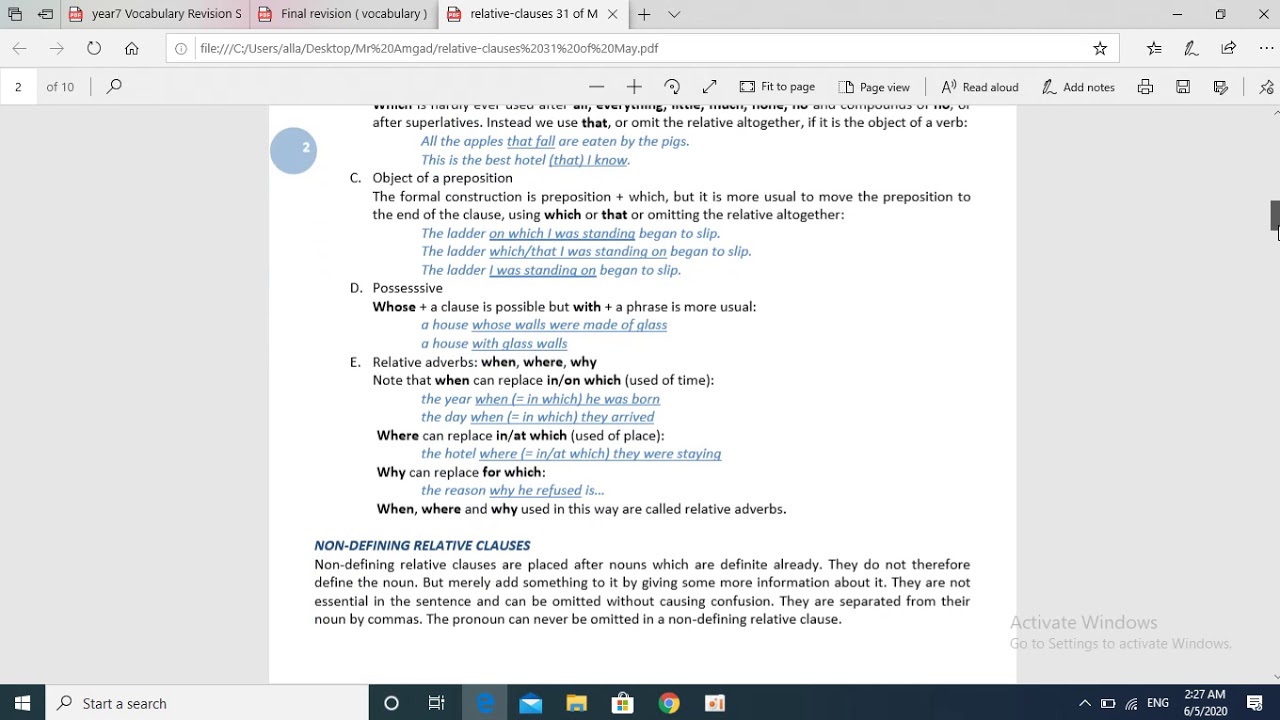This image showcases a web page screen detailing a grammatical guide on relative clauses, entitled "Relative Clauses 31 of M." The page appears to be structured like an instructional document, offering explanations and examples in a clear format.

At the top of the page, a section covers the use of relative clauses after superlatives, explaining that "that" can be used or omitted altogether if it functions as the object of a verb. Examples provided include: "All the apples that fall are eaten by the pigs" and "This is the best hotel that I know." 

Another highlighted area, labeled "Object of a Preposition," addresses formal and informal constructions. It explains that while the formal structure is preposition plus "which" (e.g., "The ladder on which I was standing began to slip"), it is more common to move the preposition to the end of the clause, allowing for variations like "The ladder which/that I was standing on began to slip" and even "The ladder I was standing on began to slip."

The document continues with detailed sections on possessives, using "whose," and relative adverbs like "when," "where," and "why," each accompanied by illustrative examples.